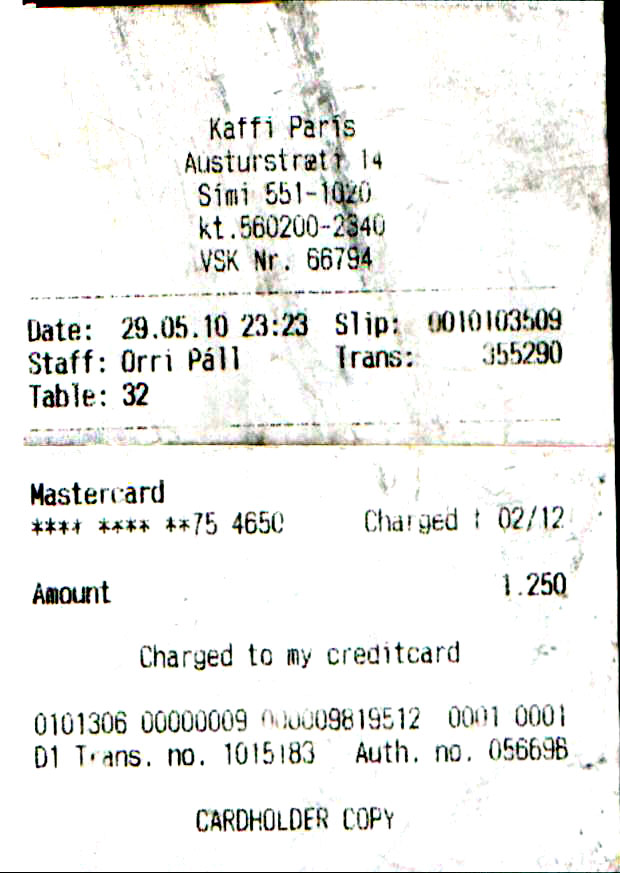The image is a black and white photocopy or scan of a receipt, which looks rough with streaks and areas that appear dirty and faded. At the very top, centered text reads, “Kaffee Paris AUSTURSTRAET 14.” Below it is the text "CIMI 555-1020" followed by "KT 560200-2340." There's a dotted line separating this information from the rest. The receipt is dated "29.05.10" at "23:23". The document includes various codes and identifiers like the slip number "001-01-03-509", staff identified as "O-R-R-I-P-A-L-L", and transaction number "355-290". It's noted that the table number is "32". The payment was processed through MasterCard, ending in "754650", with an amount that seems to be "$1,250" or a charge of "212." The term "charged to my credit card" is visible along with a bunch of faded numbers and an authorization number "05669B". At the very bottom, it states "Cardholder Copy".